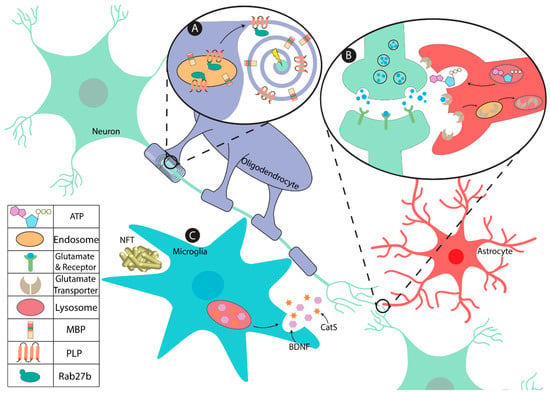This detailed and colorful scientific diagram illustrates a complex biological process within the body's cellular function system. At the center of the image, a light blue neuron, illustrated with its characteristic dendritic branches, connects towards several other cellular structures, emphasizing interaction. Below this neuron, a teal-colored microglia is shown with an outburst star shape. Adjacent to the microglia, there's a bright red astrocyte with extensive branching, distinctly visible on the top right of the diagram.

Each of these cells is connected through a series of labeled pathways indicating various biochemical interactions. The diagram features labeled elements such as BDNF, CMS, and NFT, depicted with detailed annotations. To the left side of the image, there is a key for these elements, displaying images and names like ATP, Endosome, Glutamate Receptor, Glutamate Transporter, Lysosome, MBP, PLP, and RAB27B. These components are shown in colors such as aqua, green, coral, and purple, making the diagram visually appealing and easy to navigate.

Furthermore, the accompanying table at the bottom visualizes these interactions with clear images of ATP, an endosome, a glutamine receptor, a glutamine transporter, a lysosome, MBP, PLP, and RAB27B. Dotted lines and annotations demonstrate the dynamic interactions and processes, although the specific biological process remains unidentified in the image. This diagram effectively uses color coding and detailed illustrations to convey the complex biochemical relationships within cellular processes.